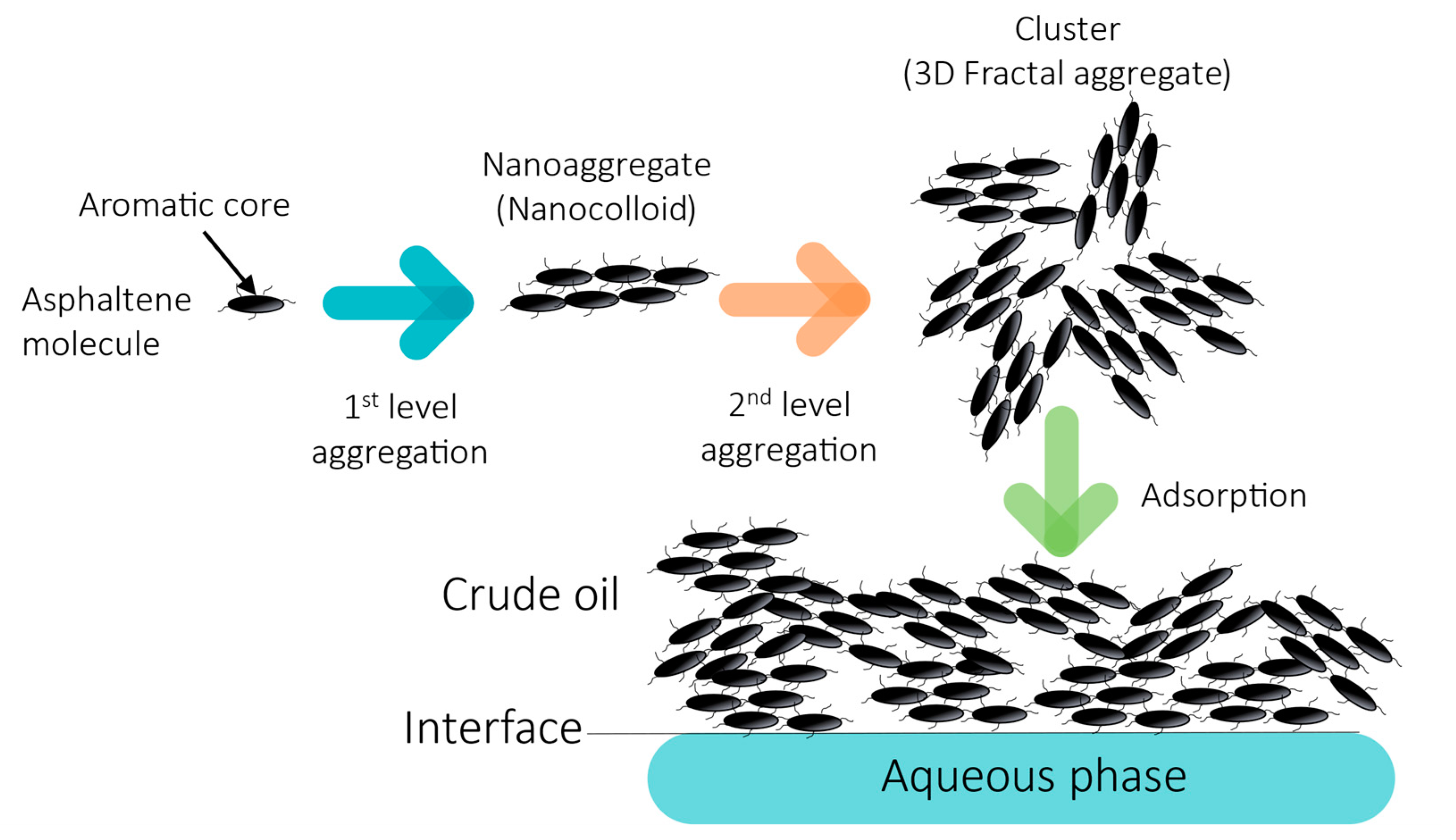This detailed diagram illustrates the sequential process of crude oil components aggregating from aromatic cores to larger structures. Starting at the top left, it displays an "Aromatic Core" labeled as an asphaltene molecule, depicted as a dot with five protruding lines. This single unit undergoes "First Level Aggregation" via a blue arrow, forming a "Nano-Aggregate" composed of six such molecular units. Progressing through an orange arrow labeled "Second Level Aggregation," these nano-aggregates cluster into a "3D Fractal Aggregate," appearing as a network or mass of interconnected units. A green arrow then indicates the transition to the "Adsorption" phase, where the aggregates further consolidate into larger masses, illustrating interaction with the crude oil interface. At the bottom, a blue bar with rounded corners labels this culminating phase as the "Aqueous Phase." Arrow annotations and color codes guide through each step, emphasizing the complexity and hierarchical aggregation from individual molecules to large clusters within the crude oil — detailing both the microscopic and macroscopic transformations.